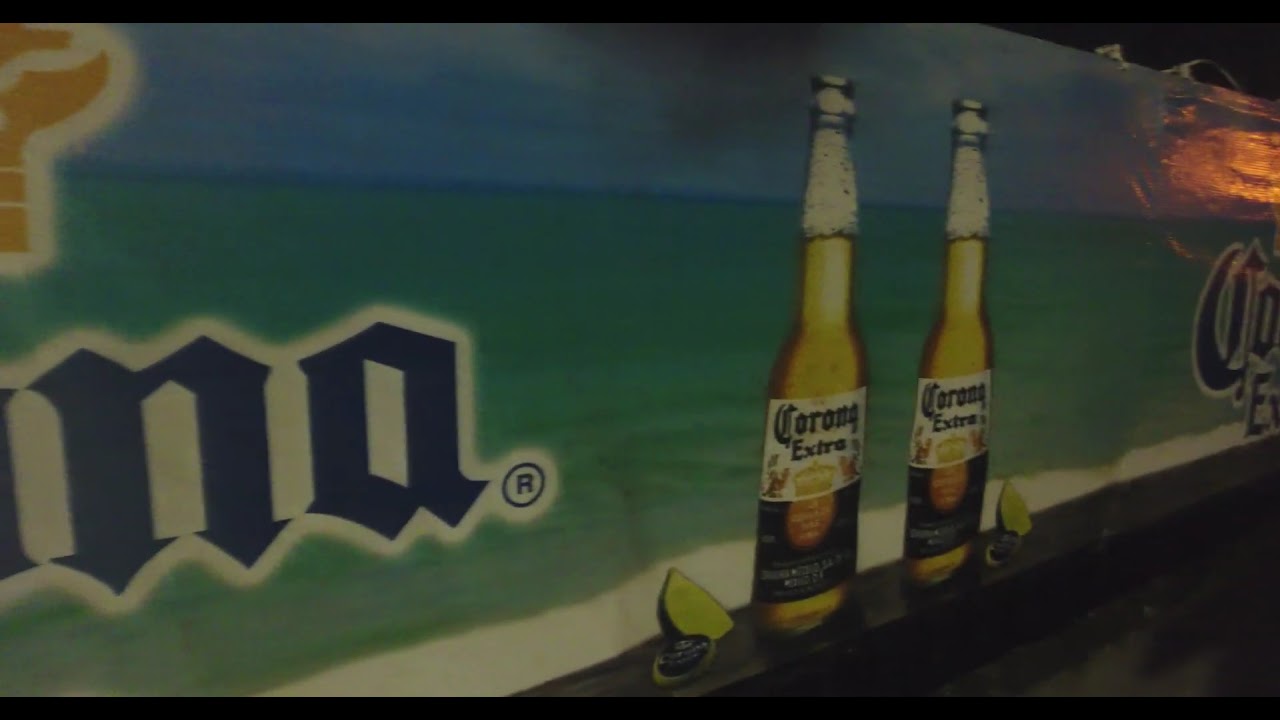The image is a close-up photograph of a billboard advertisement for Corona Extra beer, possibly situated in a dimly lit or nighttime setting. The billboard appears as though it could be on a wall, the side of a roller rink, or even the side of a six-pack box. The ground visible in the bottom right corner is shrouded in darkness, making it difficult to discern its material. 

The billboard design is split horizontally into two sections: the top third is light blue, reminiscent of the sky, while the bottom part is a lighter green, suggesting an ocean. This painted backdrop features two tall glass bottles of Corona Extra, each with a lime positioned beside it. The white Corona Extra labels are prominently displayed on both bottles, which remain unopened. 

In large blue letters, part of the brand name "Corona" is visible on the left side of the image, showing "NA." The upper right corner of the billboard is lightened, potentially by a spotlight or an intentional highlight in the advertisement design. There is also a thin black bar running horizontally across both the top and bottom of the photograph, framing the content. The overall dark ambiance around the sign underscores the focus on the brightly colored and illuminated beer bottles.